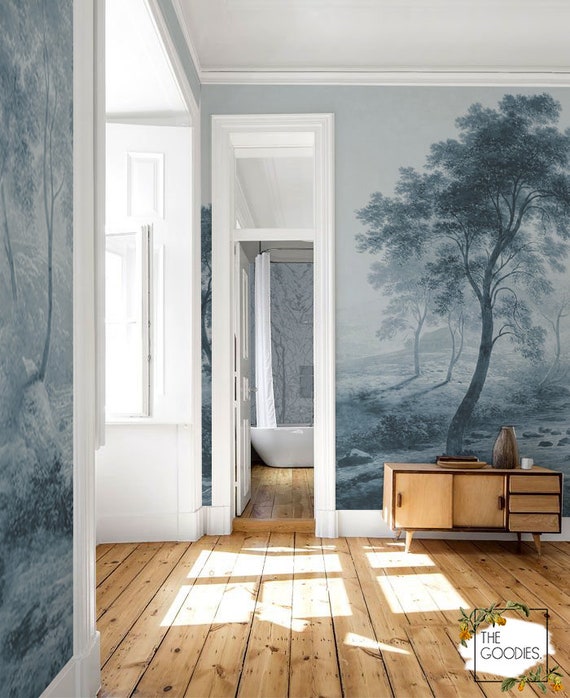The photograph captures a sun-filled interior of a very expensive house, distinguished by its unique and artistic elements. Luxurious, hand-painted murals adorn the pale gray-blue walls, depicting tranquil, pastoral scenes in an 18th-century style. The wide wood plank floors exude warmth and elegance, stretching through the visible spaces of the home.

In the bottom right-hand corner, a botanical logo reading "The Goodes" is set within a decorative box frame, likely indicating the family's name. A mid-century modern sideboard or entertainment center is notable on the right side of the image, adorned with a vase and a tray, enhancing the room's sophisticated aesthetic.

The house boasts vaulted ceilings and large transoms above the white-painted interior doors, adding to the grandeur. Crown molding, also white, complements the overall décor. A narrow hallway leads to a modern bathroom, where a white vessel bathtub and a white shower curtain come into view.

While there are some peculiar architectural features—such as a door that seems disproportionately slim for its frame and a wall that transitions abruptly from door to window—the overall scene depicts an opulent and thoughtfully designed living space that merges classical artistry with modern amenities.